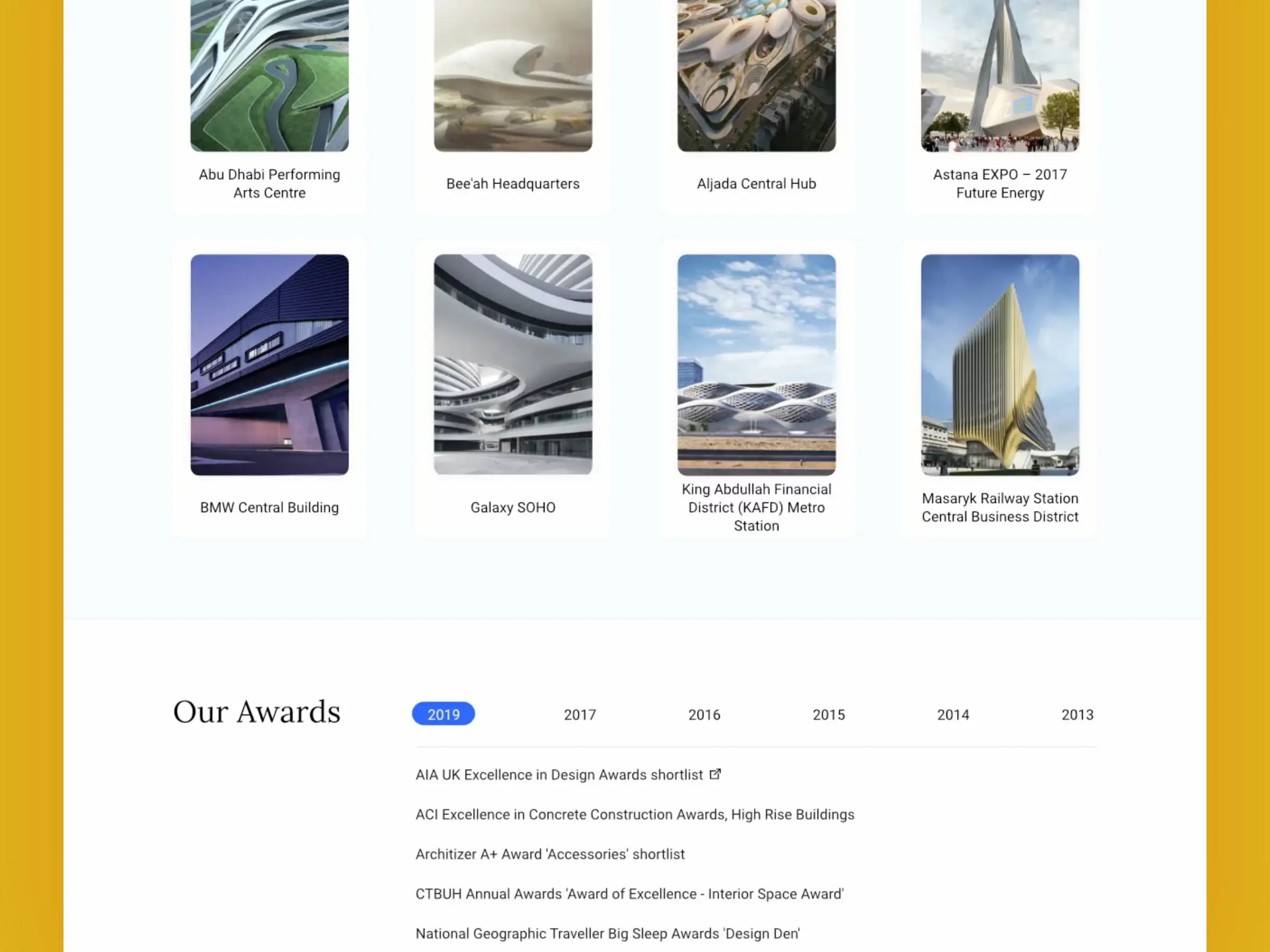The website features a white background with gold, mustard-colored bands on either side. The main section displays a grid of eight images arranged in two rows. Below the images, a blue-highlighted text reads "Our Awards 2019". Additionally, award years from 2013 to 2017 are listed, alongside the titles of various accolades: AIA UK Excellence of Design Awards Shortlist, ACI Excellence in Concrete Construction Awards, High-Rise Buildings, Architizer A-Plus Award Accessories Shortlist, CTBUH Annual Awards, Awards of Excellence, Interior Space Awards, National Geographic Traveler, and Big Sleep Awards Design Den.

The images themselves are cut off halfway, and each has a caption with notable architectural projects. The top row includes:
1. ABU-DHABI Performing Arts Center
2. BEE-AH Headquarters
3. AJADA Central Hub
4. IASTANA Expo 2017 Future Energy

The bottom row features:
1. MBMW Central Building
2. Galaxy SOHO
3. King ABULA Financial District
4. Metro Station